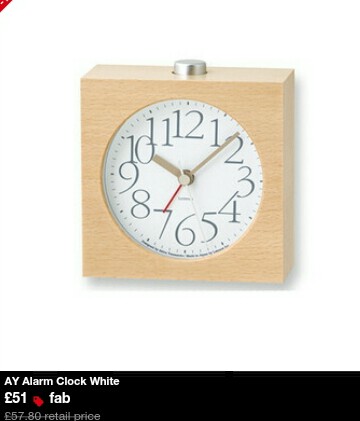The image is an advertisement showcasing a square-shaped alarm clock encased in light beige wood. The clock features a white circular face with bold black numbers ranging from 1 to 12, except for a slight overlap where the numbers 10 and 11 touch. The clock boasts a thick brown hour hand, a thin brown minute hand, and two additional rods—a red second hand and a white indicator. The clock's frame has a polished and smooth finish with a small silver button on top. The current time displayed is 10:09. At the bottom of the image, the text reads "AY Alarm Clock White," followed by a price tag showing "£51" marked with a red label stating "FAB," with a retail price of "£57.80" underneath.